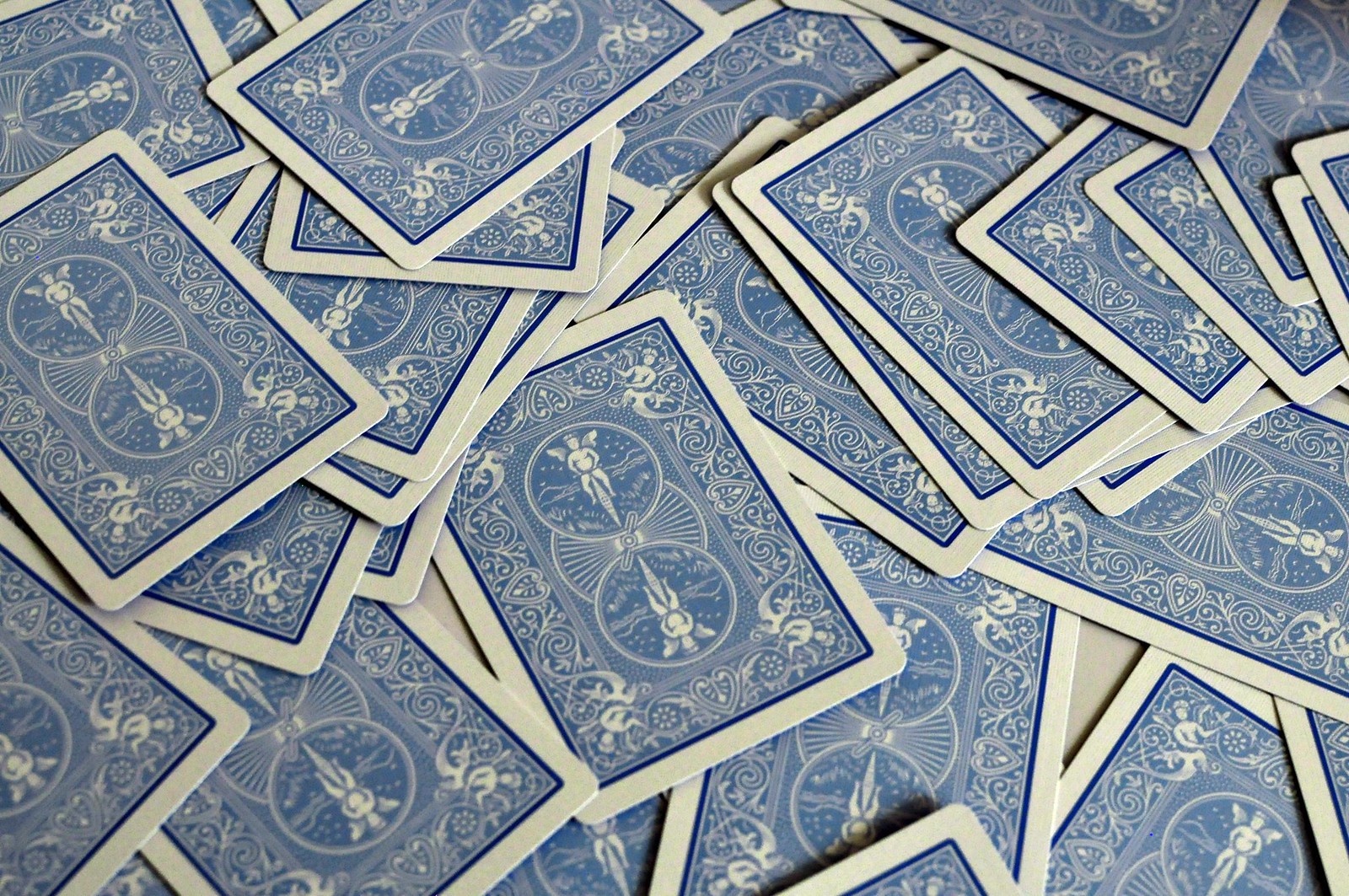In this image, a collection of playing cards is scattered across what appears to be a white table. The cards are all facing downward, showcasing their intricate blue backs instead of their numbered sides. Each rectangular card features a prominent blue outline. Inside the outline, angelic figures adorn the design. 

At the center of each card, there are two circles, each containing an angel. These angels are depicted with spread wings and legs, with a diamond pattern placed underneath their legs for additional detail. A third, hidden circle with striped patterns is situated between these two central angels.

In the corners of the cards, additional angels are etched, each pointing in specific directions. The card backs are further embellished with elaborate heart motifs and swirling designs, adding to the overall complexity and beauty of the artwork.